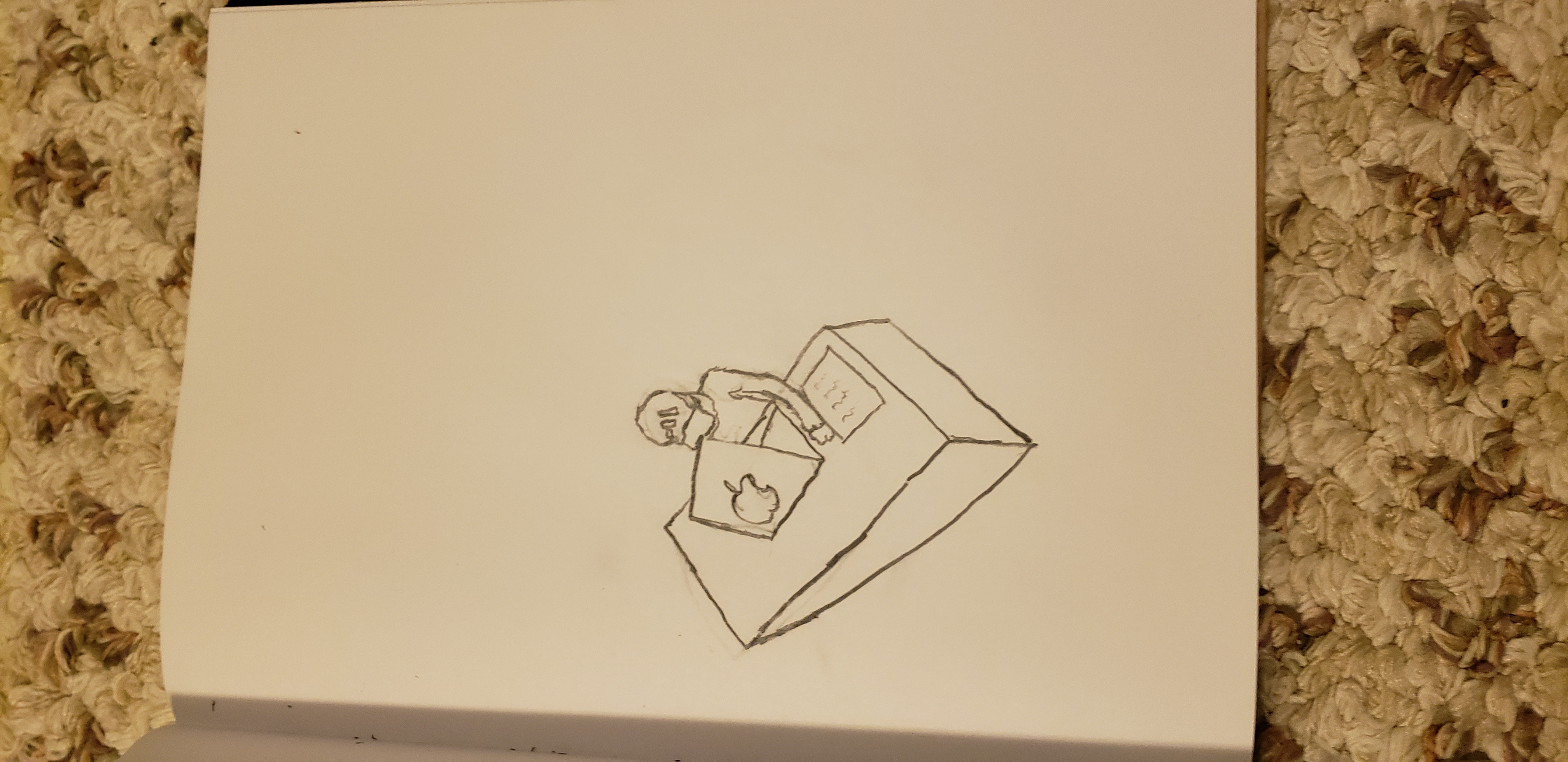The image showcases a detailed pencil drawing on a sheet of paper positioned sideways within an open notebook, placed on a white and brown, thickly textured carpet, possibly Berber. The carpet's surface is characterized by its knotted texture, contributing to its distinctive pattern. The drawing on the paper features a desk depicted as a rectangular cube, complete with a smaller rectangle symbolizing a sheet of paper with scribbled lines. Additionally, there's a small figure wearing a hat, seated before a laptop that prominently displays an apple logo on its back. The meticulous details in the drawing and the texture of the surrounding carpet add a rich context to the scene.